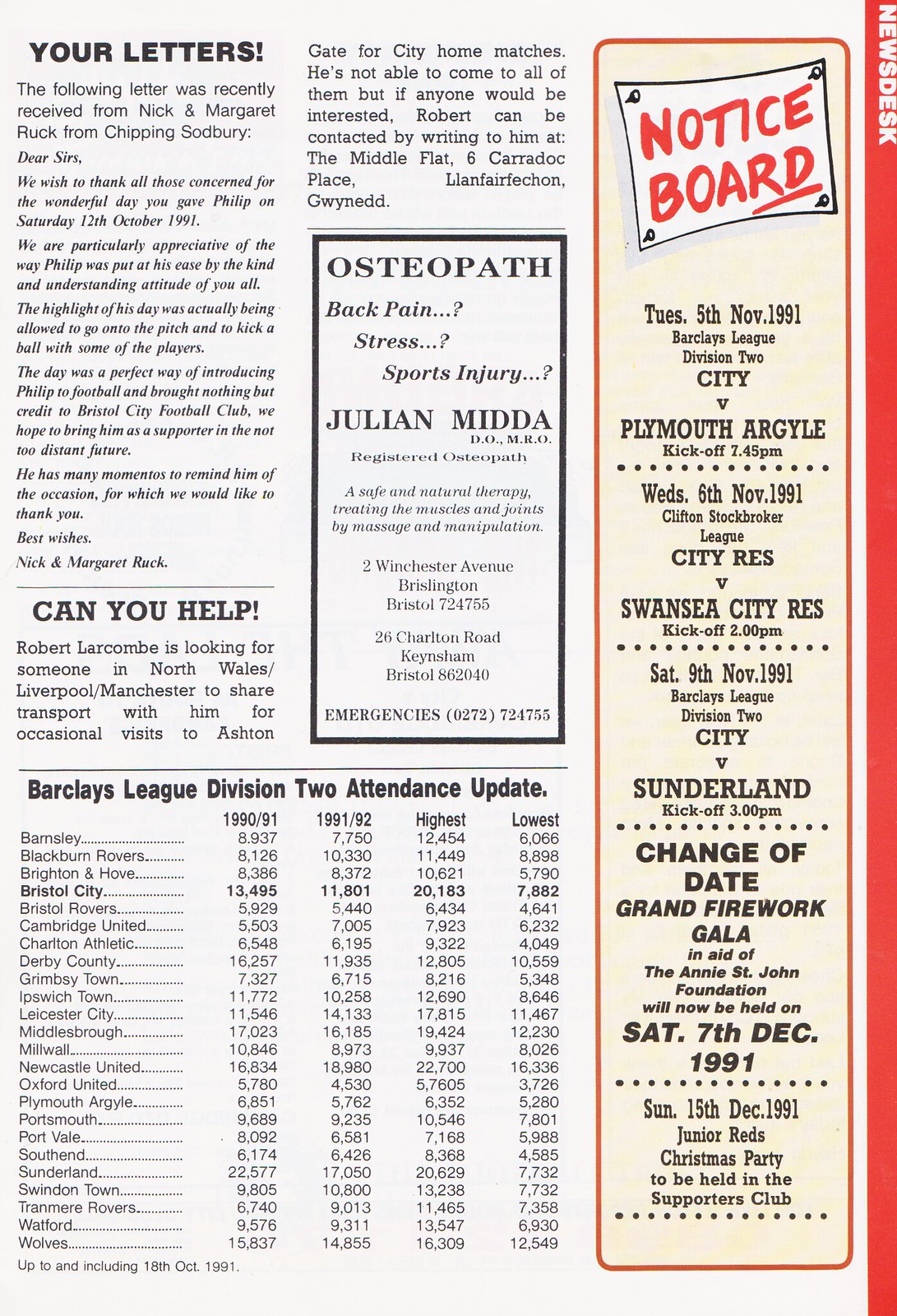The image is a detailed black and white printed page from a vintage football club program, prominently featuring elements in red and cream for visual emphasis. In a portrait layout, the top left corner displays a section titled "Your Letters" in bold, followed by a series of letters from subscribers, including one from Nick and Margaret Ruck from Chipping Sodbury. Beneath this, a smaller subsection titled "Can You Help!" includes a brief paragraph essaying assistance.

On the right side of the page, encased in a red-bordered column on a cream background, there is a "Notice Board" header in red lettering with contact details and dates for various 1991 events, such as fireworks on Saturday, 7th December 1991. The bottom section contains a prominently displayed "Barclays League Division 2 Attendance Update" with intricate statistics about team attendances over different years, specifically highlighting 1990 and 1991 figures. Adjacent to this section is an advertisement for osteopathic services by Julian Mida, DO, MRO, specializing in back pain, stress, and sports injuries. Further adding to its character, a vertical red band labeled "News Desk" in white letters runs down the right side of the page.